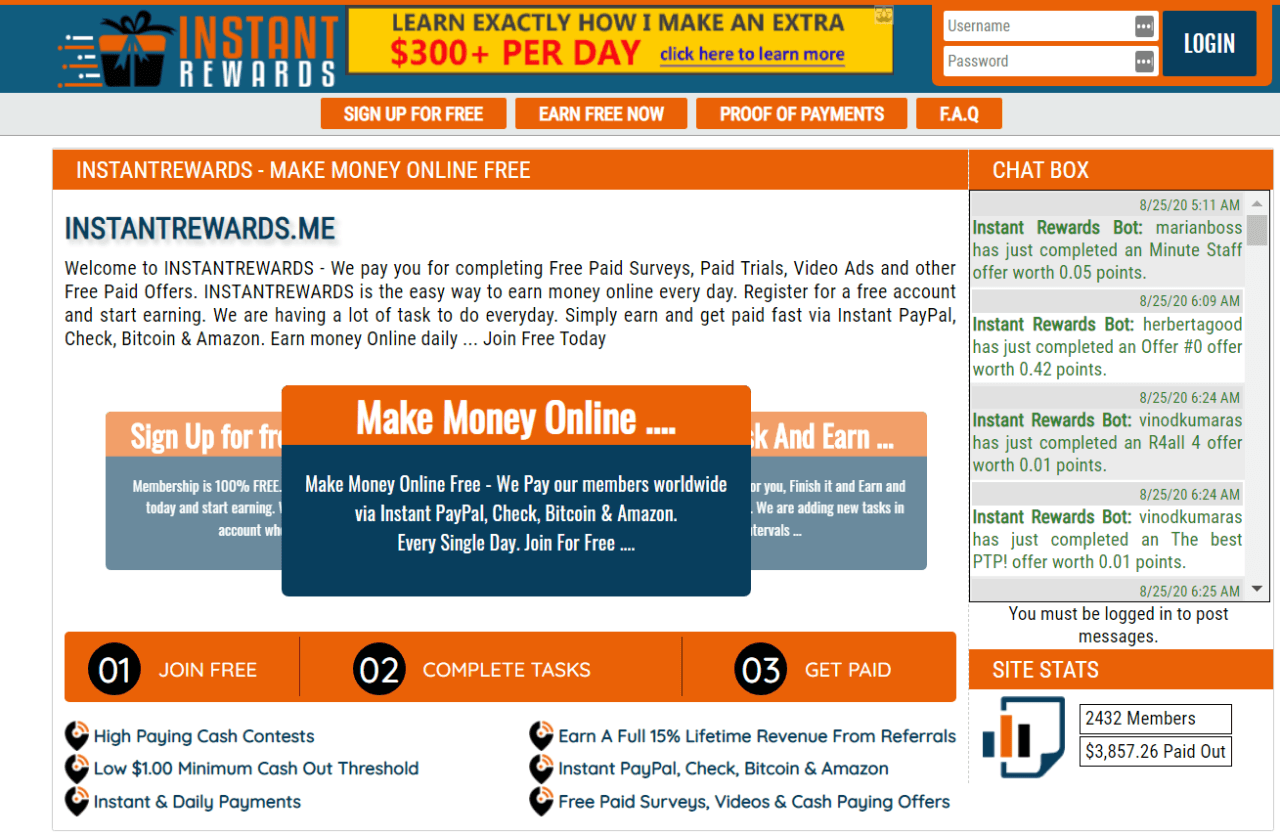The webpage entitled "Instant Rewards" is displayed prominently with repetitive text at the top, emphasizing "Instant Rewards" and "make money online free" through rewards.me. Below the header, there's a large descriptive section that welcomes users to Instant Rewards, a platform that pays for completing free paid surveys, trials, video ads, and other offers. The site falls under the category of get-paid-to websites or survey sites and has a visually chaotic and unappealing design, cluttered with various elements.

In the foreground, a prominent pop-up invites users to make money online, highlighting that the platform pays members worldwide every day via Instant PayPal, Check, Bitcoin, and Amazon, and emphasizes that joining is free. The overall color scheme features a white background with an abundance of orange accents.

On the right side of the page, there's a chat box run by the Instant Rewards bot, which displays recent user activities such as "Marian Boss has just completed a MinuteStaff offer worth five cents or 0.05 points." At the top right corner, there's a login button, and a large banner ad spans the top of the page.